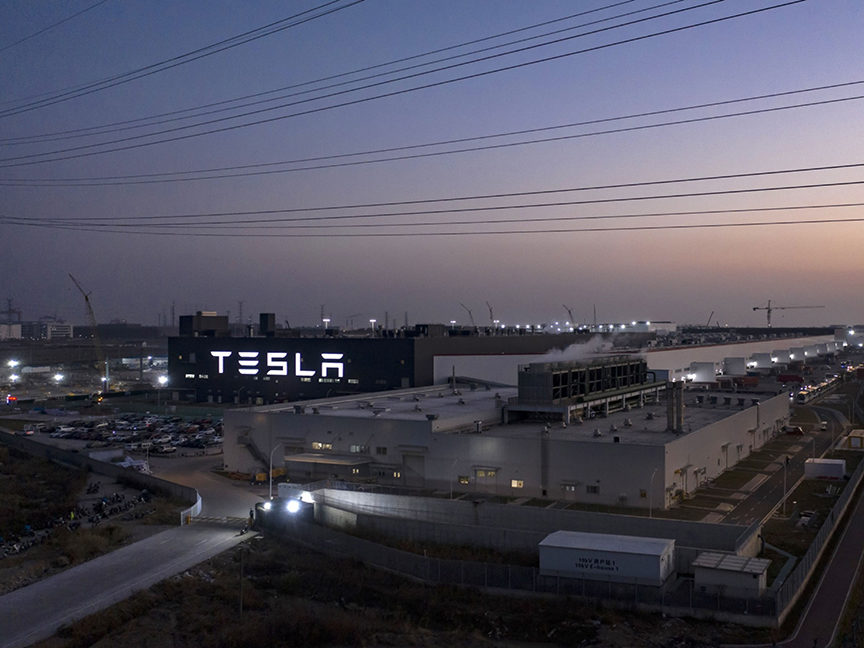This photograph captures the expansive Tesla car plant at dusk, marked prominently by an illuminated white "Tesla" sign adorning the front of the building. The scene is set during sunset, casting an array of purple and orange hues across the sky, lending a serene yet industrial ambiance to the image. The vantage point suggests the picture was taken from a distance, emphasizing the scale of the facility. Visible steam or smoke wafts from air-conditioning units atop the building, which is a central, gray structure within a larger compound-like area. A full parking lot suggests workers have not yet left for the day. In the background, streetlights and power lines are seen, contributing to the factory's isolated yet industrious atmosphere. A security gate with a brightly lit security shack stands at the compound's entrance, adding to the detailed tableau of a busy and secured manufacturing environment.